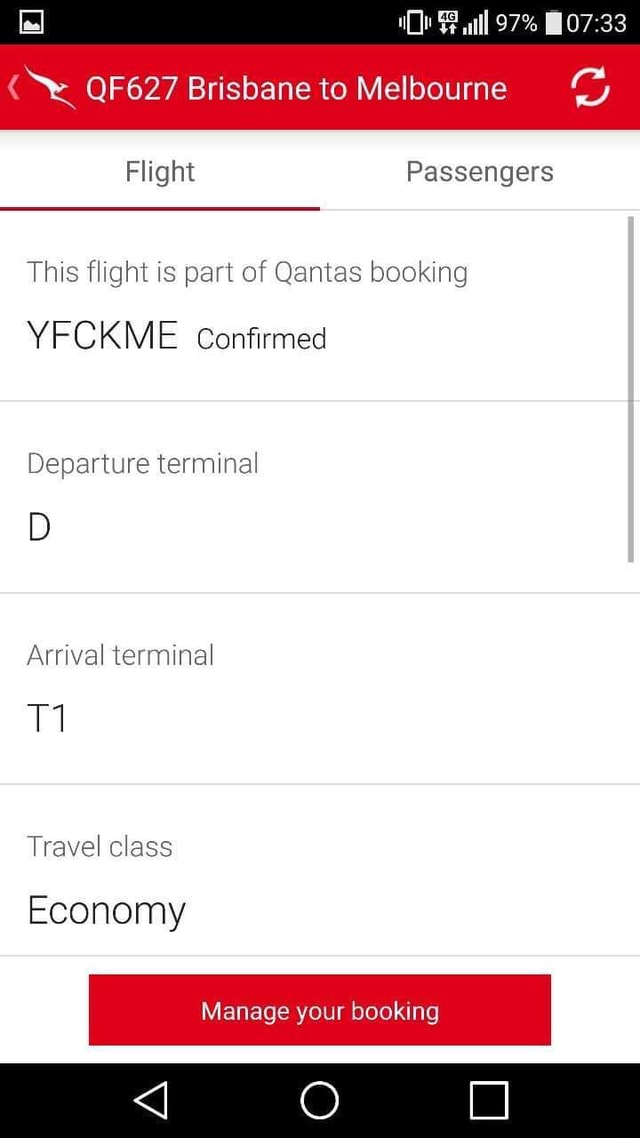The image is a screenshot of a flight booking webpage. At the top, the text displays "QF627 Brisbane to Melbourne," indicating the flight number and route. It further states "Flight" on one side and "Passenger" on the other, splitting the information sections. The text confirms that the flight is part of a Qantas booking with the reference code "YFCKME" and it mentions that the booking status is confirmed. 

For more details, it specifies that the departure will take place at Terminal D, and the arrival is scheduled at Terminal T1. The travel class mentioned is Economy. Below these details, there are options to "Manage Your Bookings," possibly allowing changes or viewing more details about the reservation.

Additionally, at the bottom of the page, there are phone icons, likely suggesting contact options or customer service. Other navigation elements include a homepage button, a back button, and a tabs button, which are positioned at the very bottom of the page, facilitating easy access and navigation for the user.